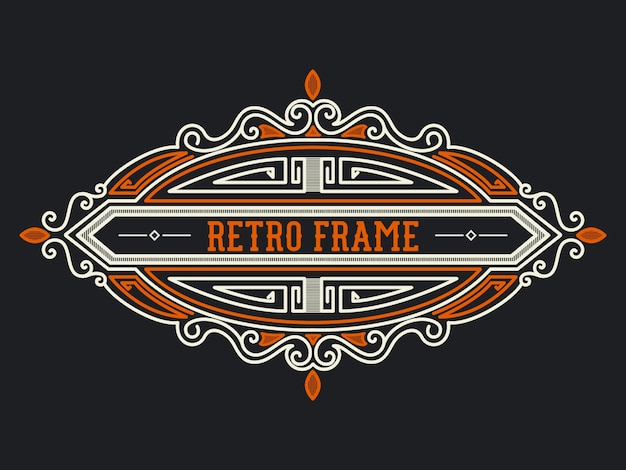Set against a completely black background, this detailed illustration features an oblong, somewhat football-shaped emblem predominantly colored in orange, black, and cream. The central part of this emblem includes a long, narrow bar with a black background, showcasing the text "Retro Frame" in bold, all-capital, orange letters. Encircling this central bar are intricate decorations, including brownish-orange decorative ovals positioned strategically at the top, bottom, left, and right corners. The emblem is adorned with additional black and white filigree and various accents that enhance its vintage aesthetic. The entire illustration, which appears computer-generated or meticulously drawn on a tablet, exudes a retro charm through its multicolored, ornate design.